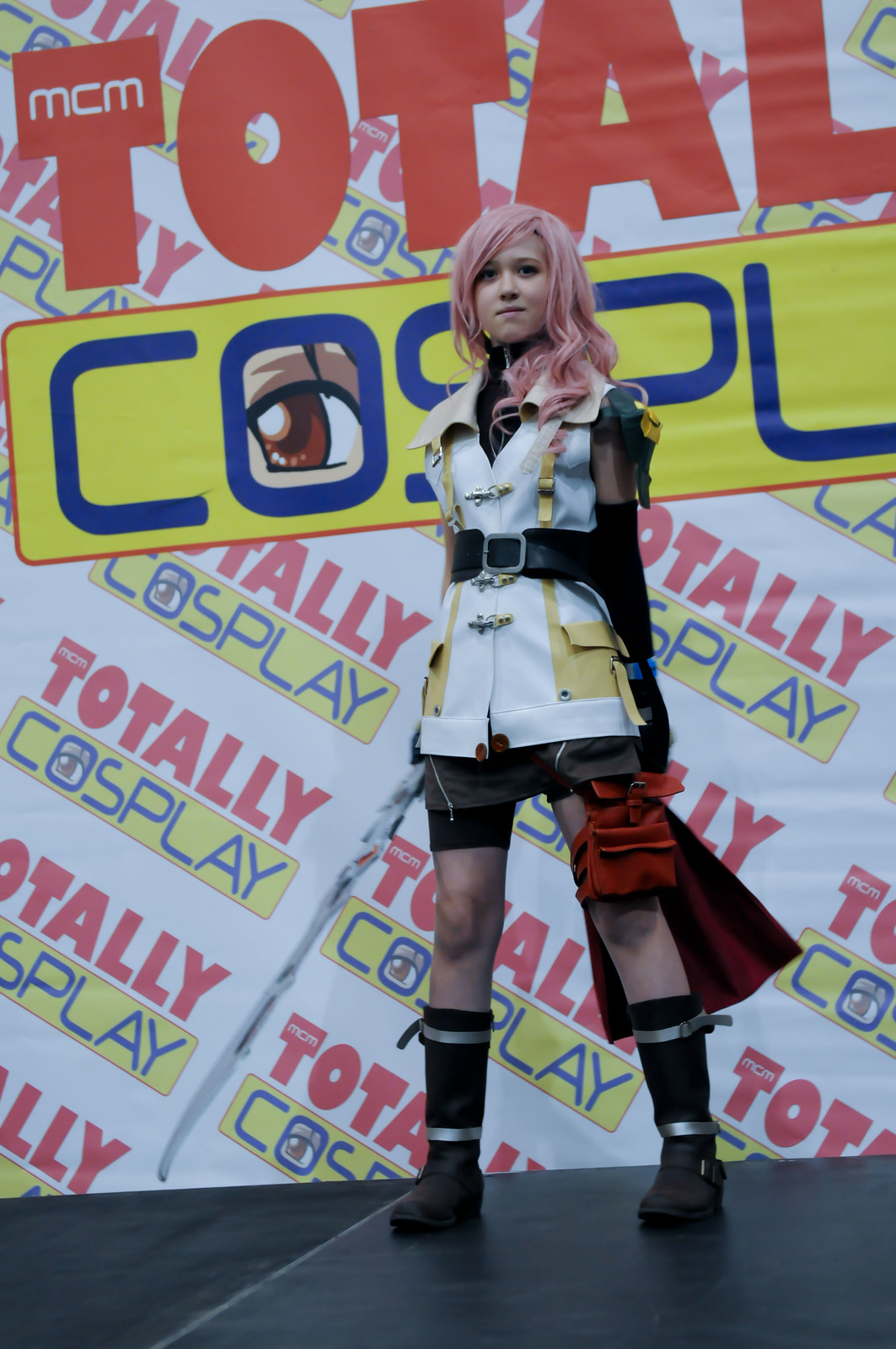In this image, a woman with light pink hair stands confidently on a black stage. Behind her is a white backdrop patterned with logos that read "Total Cosplay" in red, yellow, and blue. She is outfitted in an elaborate cosplay costume, featuring tall black boots adorned with thin silver straps, which reach her mid-calf. Her dark shorts extend to mid-thigh, complemented by a vibrant red bag strapped around one thigh. Over this, she wears a distinctive sleeveless white and yellow vest-like coat, cinched with a large black belt. Her ensemble includes long black gloves, a brownish-tannish short skirt, and a hint of black leggings underneath. She also holds a small red purse in her left hand and wields a long silver sword, enhancing her character's dynamic presence. She is smiling, and the logos behind her repeat in a diagonal pattern, setting the scene for this lively cosplay presentation.